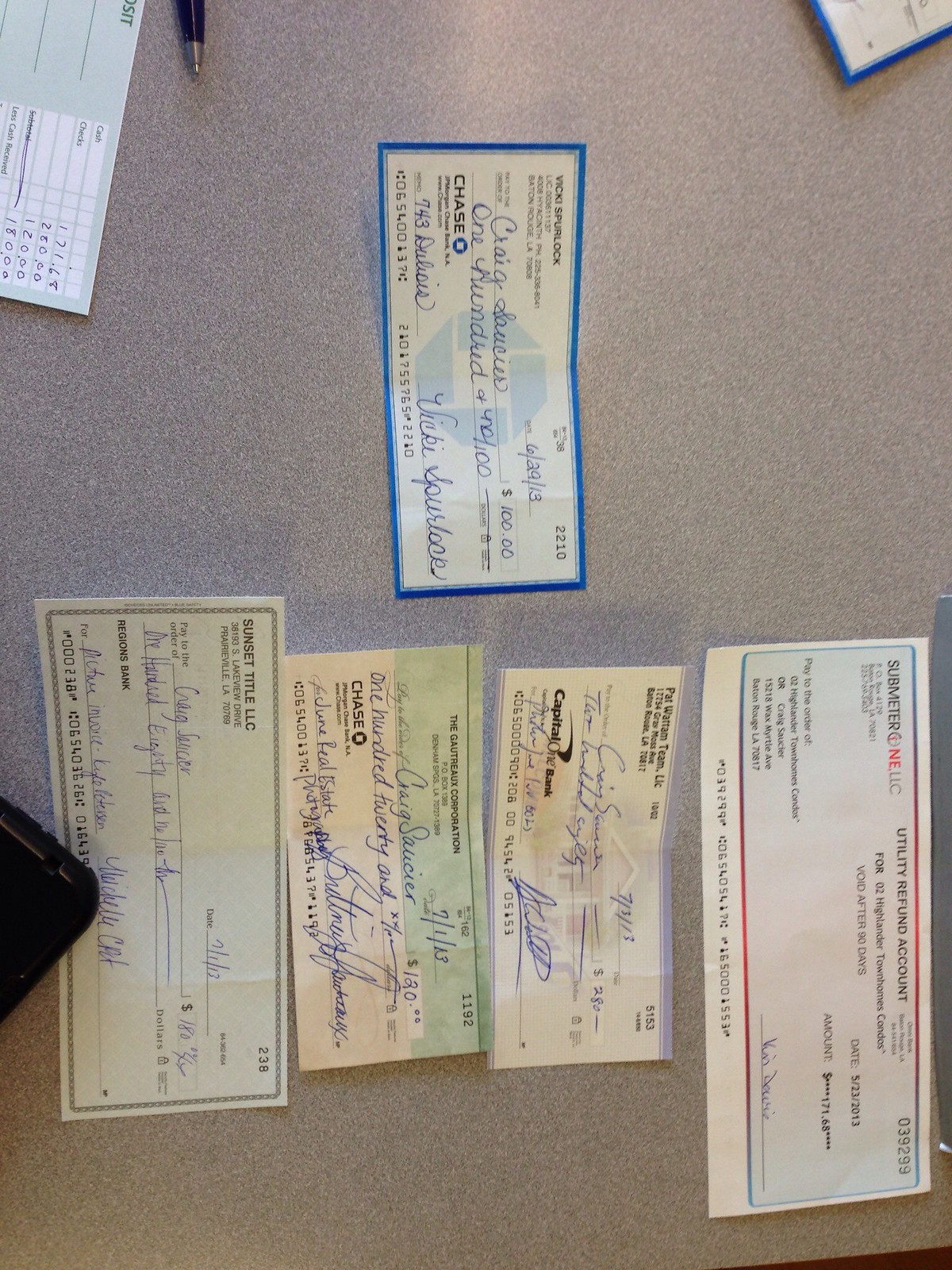The photograph, taken from an overhead angle and displayed sideways, shows five distinct checks laid out on a desk. Each check is addressed to different individuals and written with various amounts in blue pen. On the left side of the image, there is a black pen, a check register book in the upper left corner, and another piece of paper whose purpose is unclear. The checks include ones from Chase Bank, Capital One Bank, and companies like Submeter LLC. Specifically, one Chase Bank check is made out to someone named Craig for $100. The checks are densely packed with text and details, capturing a snapshot of diverse financial documents.